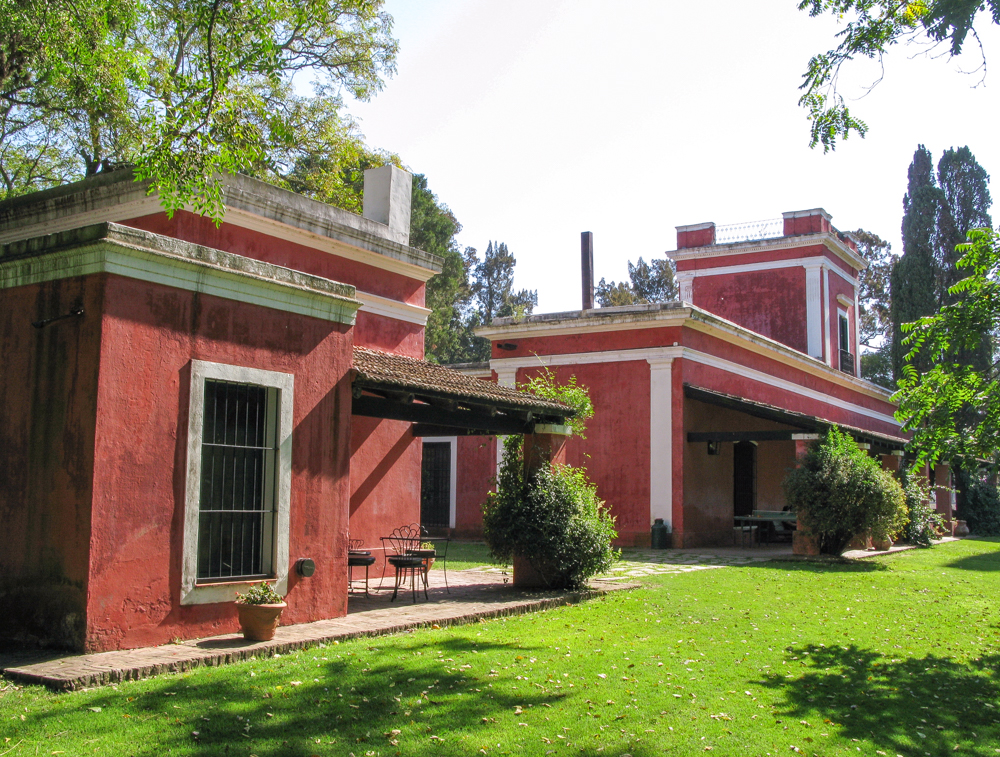This photograph captures a picturesque scene of two antique South American-style buildings set on manicured grounds. Both structures are constructed with a distinctive pinkish-red plaster and adorned with white trim, exuding an old-world charm.

The building on the left is a quaint one-story structure featuring a charming portico at its front. The portico, covered by a thatched roof, is supported by pillars entwined with lush greenery. Beneath the portico, a wrought iron bistro table invites visitors to sit and enjoy the serene surroundings. A large barred window graces the front facade, adding to the building's rustic appeal.

The building on the right is more imposing, viewed at an angle to reveal a spacious open area beneath its portico. This space is furnished with multiple tables and illuminated by overhead lighting, suggesting a communal or dining area. A striking feature of this building is its central tower, which boasts a window with a black wrought iron Juliet-style balcony. Atop the building, a widow's walk provides a panoramic vantage point, hinting at the building’s grandeur.

Both buildings are set against a backdrop of lush green lawns and surrounded by a variety of trees and plantings, creating a vibrant and inviting atmosphere. The overall scene is a harmonious blend of architectural beauty and natural splendor.